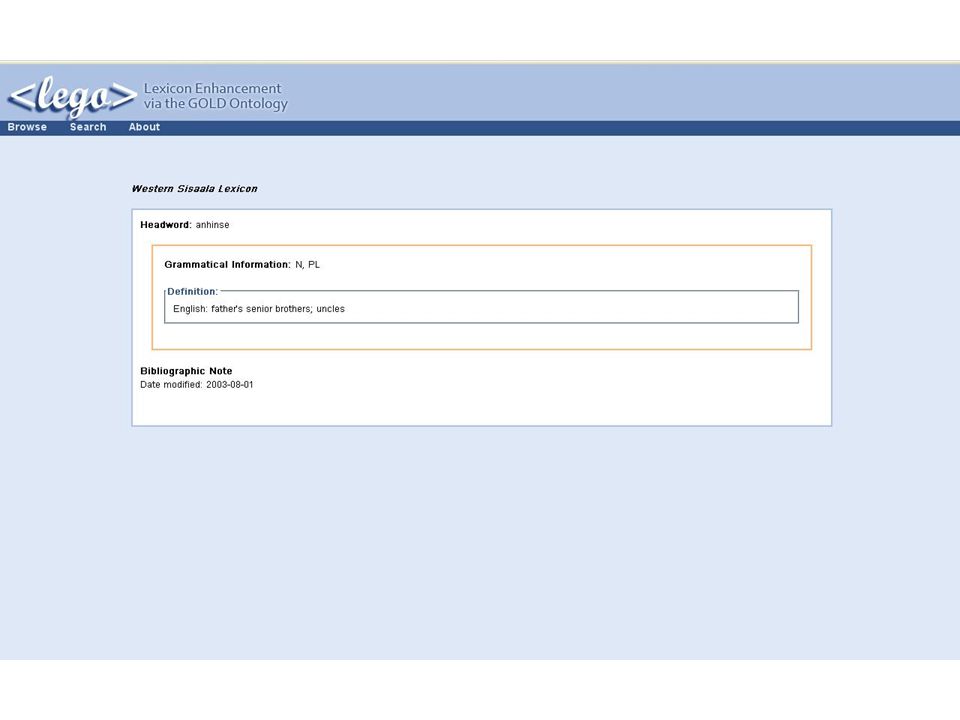This is an image of a document from a company named Lega, set against a blue background. The header features the company's name, possibly "Lego," but it reads "Lega," accompanied by the phrase "Lexicon Enhancement via Gold Ontology." Below this header is a dark navy blue box containing three clickable options: "Browse," "Search," and "About." Directly beneath the box, the document lists the entry for "Western Sizzla Lexicon" under the heading "Hedward" and subtitled "East." Here, grammatical information is provided as "N, PL," indicating that the term is a plural noun. The definition given is "Fathers, Senior Brothers, or Uncles" in English. The entry also specifies the date it was last modified: "8-1-2003."